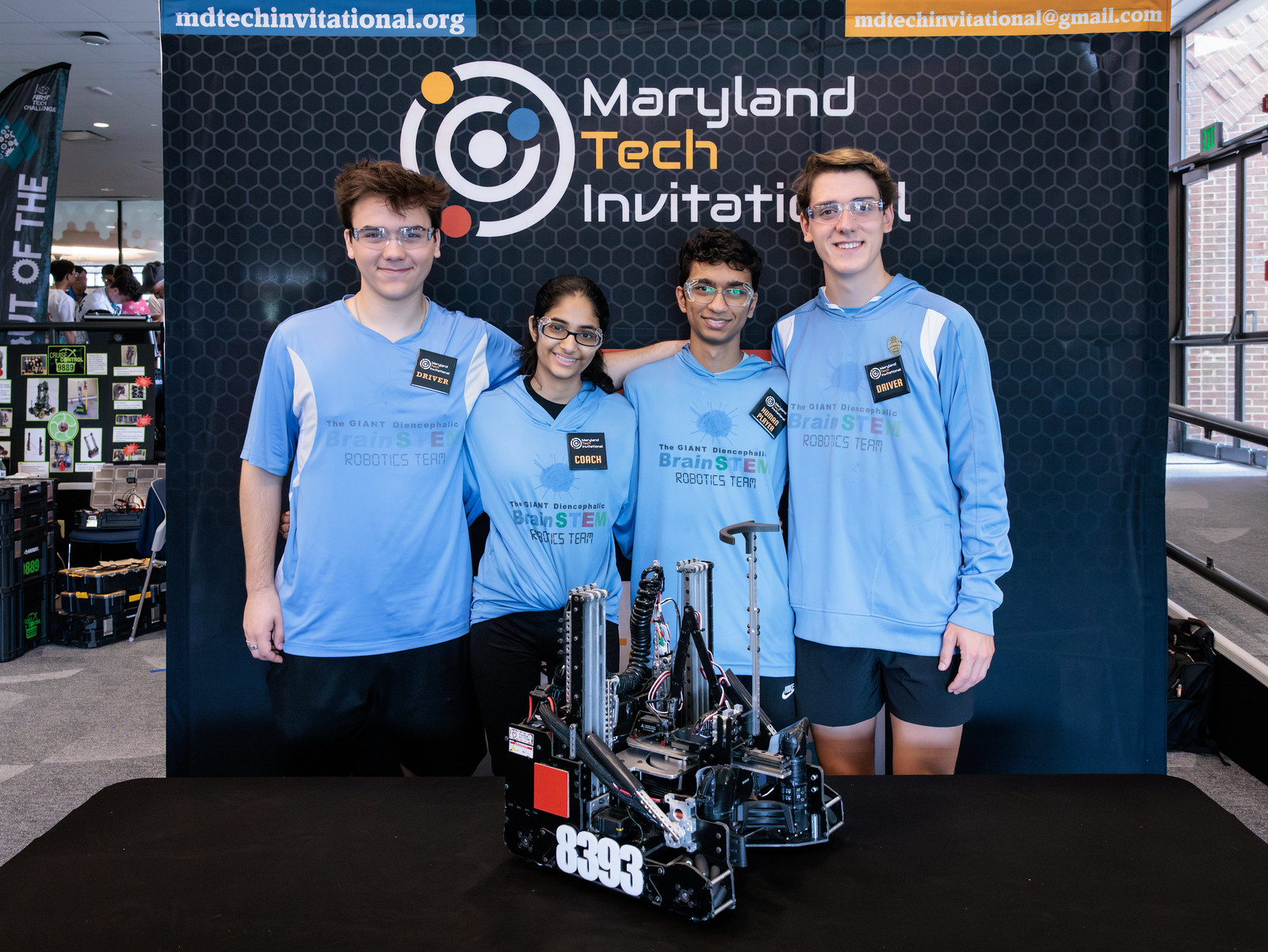Four students from the Brain STE Robotics Team, known as "The Giants," pose for a photograph at a tech exhibition. They stand in front of a dark backdrop adorned with a honeycomb pattern at the top. The backdrop prominently features the text "mdtechinnovational.com" and "Maryland Tech Innovational" on the top left, alongside white eccentric circles filled with smaller yellow, red, and blue circles. On the top right, the backdrop reads "mdtechinnovational.com."

The team members, all clad in matching blue merchandise bearing the team's name and "Brain STE Robotics Team," are organized as follows: on the left, a white male with brown hair and black pants wearing a name tag labeled "Driver"; next to him, an Indian girl with black hair and a "Coach" name tag; followed by an Indian boy identified as "Human Player"; and finally, another white male with brown hair and a "Driver" name tag. Centered in front of them on a black table is the impressive robot they created.